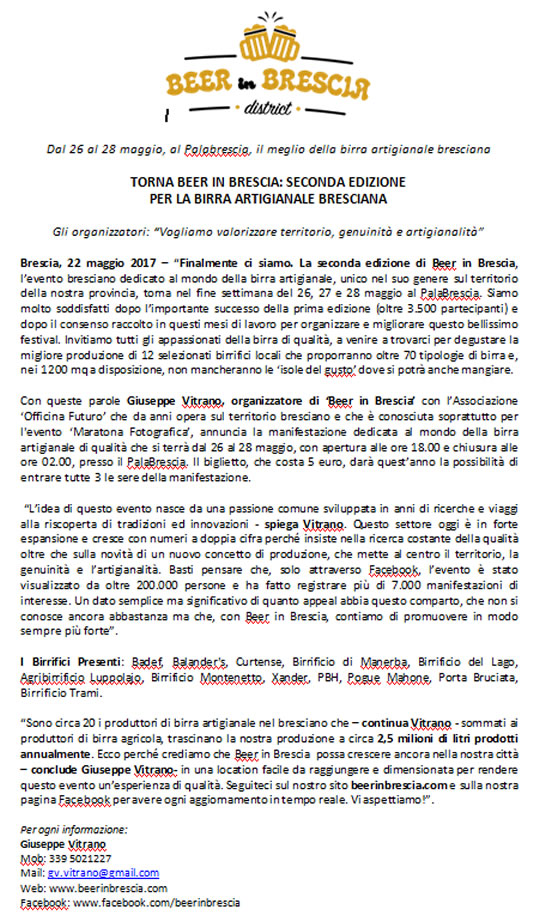The image is a black and white document with a white background, formatted in a portrait orientation and featuring spot color illustration at the top. The top of the image showcases two illustrated gold beer mugs clinking together, accompanied by a black splash overhead and a horizontal black line on each side. Below the illustration, in bold gold letters, it says "Beer for Brescia" in all caps. The word "District" appears below in a black scripted font. 

Further down, there is text written in Italian, starting with the line "Dal 26 al 28 Maggio al Palo Brescia il Meglio della Biro Artegnale Bresciana" followed by larger text stating "Torna Beer in Brescia: Seconda Edizione per la Bira Artegnale Bresciana." The document then provides five paragraphs of additional text in Italian. At the very bottom left-hand corner, contact information is provided for Giuseppe Vetrano, including his mobile number, email, web address, and Facebook address. Certain words in the text are underlined in red as if corrected by auto-correct. The overall style resembles a black and white newsletter with selective spot color accents.